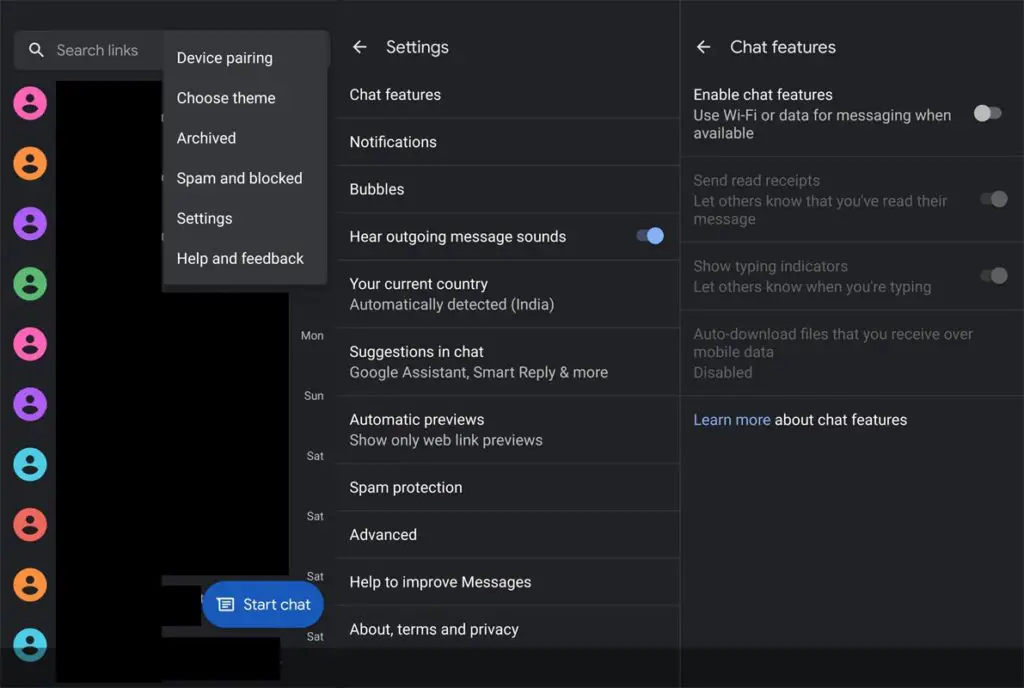This horizontal image captures a user interface on a computer or smart device, highlighting various settings and options. The background transitions from a jet black on the far left to a dull black or dark gray, creating a visual contrast.

In the upper left-hand corner, the interface offers several links for navigation, including "Device Pairing," "Choose Theme," "Archive," "Spam and Block," "Settings," and "Help and Feedback." Adjacent to these links, a vertical row of colored profile picture icons is visible, featuring hues such as pink, orange, purple, green, pink, purple, teal, red, orange, and teal.

Centrally located within the image, a detailed settings menu is displayed. It includes options for "Chat Features," "Notifications," "Bubbles," "Outgoing Message Sounds" (currently toggled on), "Your Current Country," "Suggestions in Chat," "Automatic Previews," "Spam Protection," "Advanced Settings," "Terms," and "Privacy."

The right-hand side of the image focuses on "Chat Features." Users have the option to enable these features, though it is presently toggled off. Additional options, such as "Send and Receive Read Receipts" and "Show Typing Indicators," are not available. The "Auto-Download Files Over Mobile Data" option is disabled. Users can click to "Learn More About Chat Features" for further information.